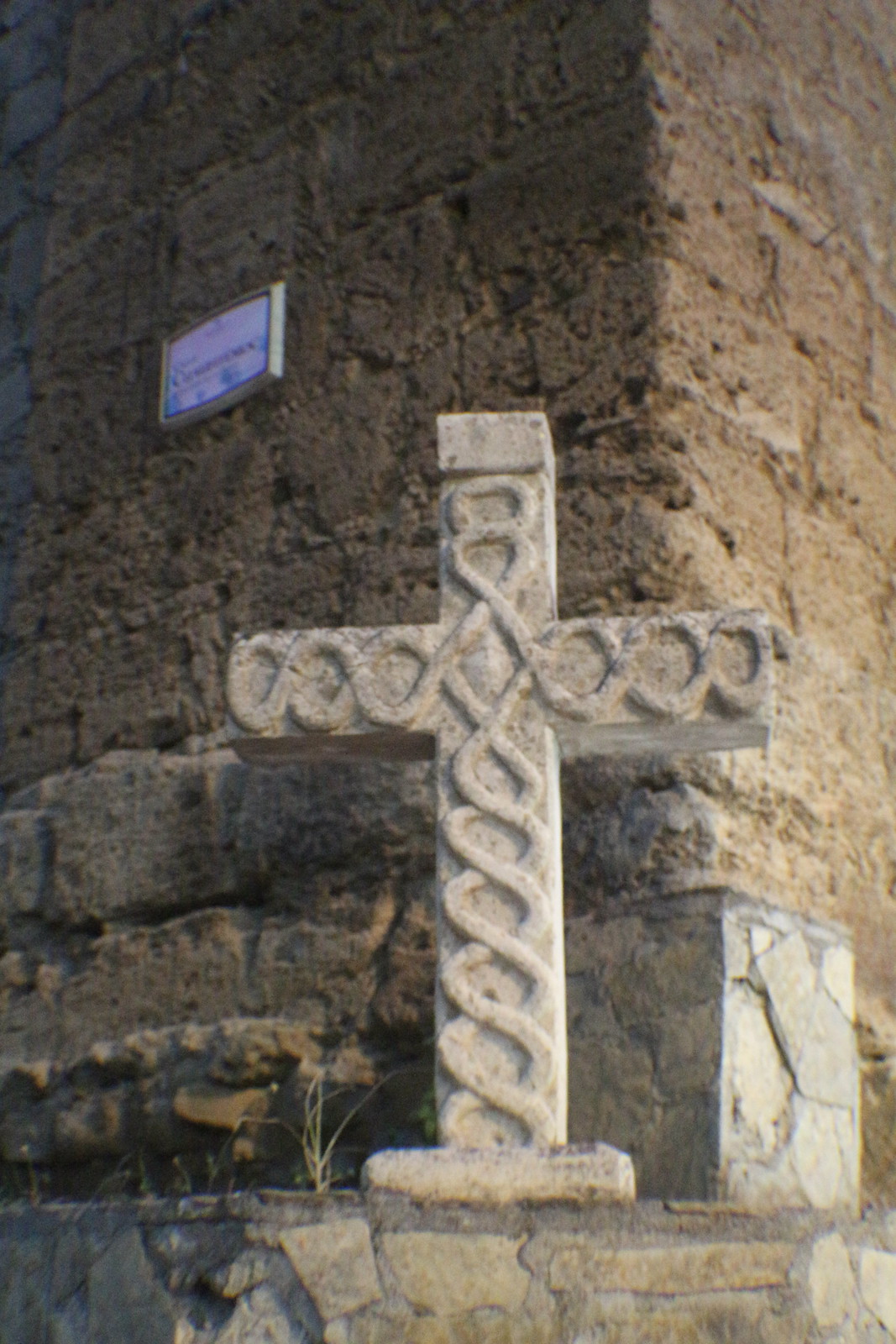The photograph depicts a carved, T-shaped stone cross prominently positioned on a stand made of mortared, irregular-shaped stones. The cross, light brown or tan in color, showcases a smooth surface with a detailed, curving, swirling helix pattern running along its front. This intricate design, resembling interwoven figure-eights, forms a diamond shape at the intersection of the lines, giving a three-dimensional, embroidered look carved from the same stone. Behind the cross stands a heavily worn, eroded stone building, characterized by its tan color and marked with numerous holes and pit marks indicative of significant weathering. The building's stone wall at the top is brown, featuring a small, gold-framed rectangular plaque with unreadable black and blue text on a white background. The entire scene is captured in a vertical rectangular frame, cutting off the base of the cross’s stand, emphasizing the aged and historical aura of the setting.